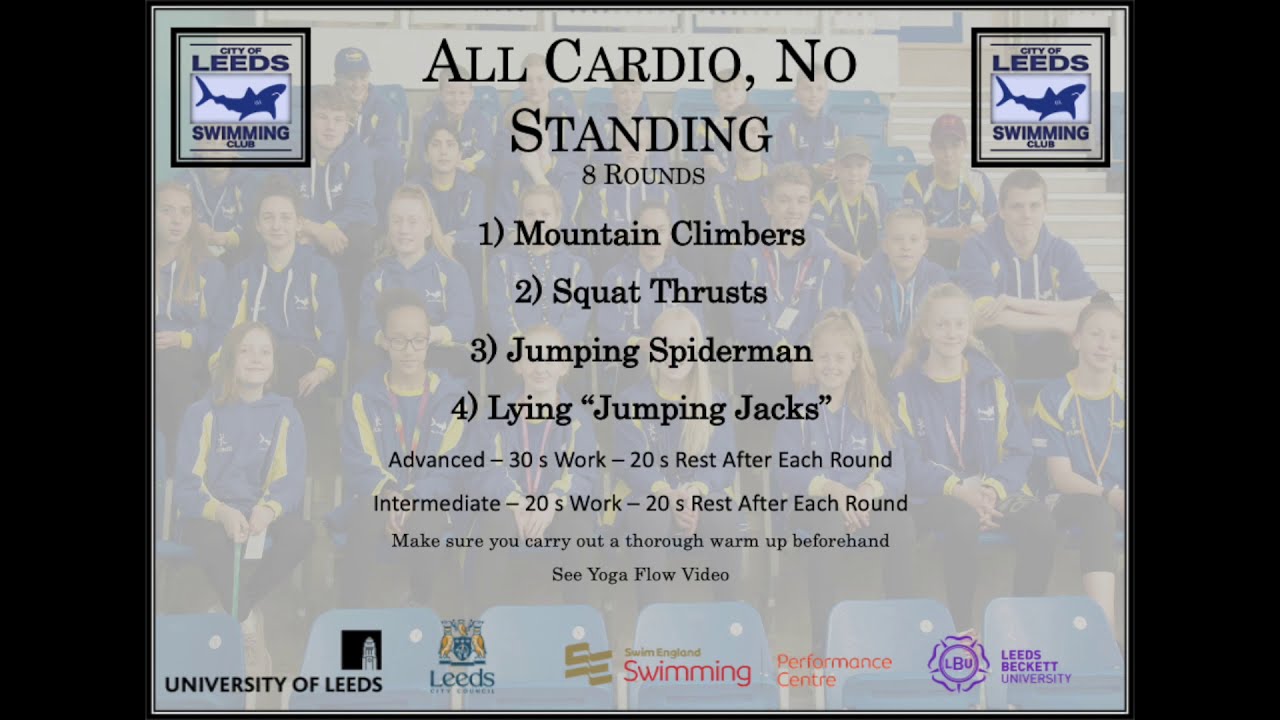The image showcases a slide for a presentation, likely related to the City of Leeds Swimming Club. At the top left and right corners of the slide, there’s the club’s logo, which includes a small blue shark encircled by the text "City of Leeds Swimming Club." The background features a muted and almost transparent image of a sports team, presumably the City of Leeds swimming team, consisting of both boys and girls in blue and yellow uniforms seated in bleachers.

The central, black, center-aligned text outlines a cardio workout routine titled "All Cardio, No Standing, Eight Rounds." The specific exercises listed are:
1. Mountain Climbers
2. Squat Thrusts
3. Jumping Spiderman
4. Lying Jumping Jacks

Advanced participants are to perform 30 seconds of work with 20 seconds of rest after each round, while intermediate participants perform 20 seconds of work with an equal rest period. A note emphasizes the importance of a thorough warm-up, directing participants to a yoga flow video for guidance.

At the bottom, logos of supporting organizations are displayed: University of Leeds, Leeds City Council, Swim England Swimming, The Performance Center, and Leeds Beckett University.

In summary, this detailed and informative slide serves as a visual aid for a structured cardio workout, likely used in a training session or presentation for the members of the City of Leeds Swimming Club.